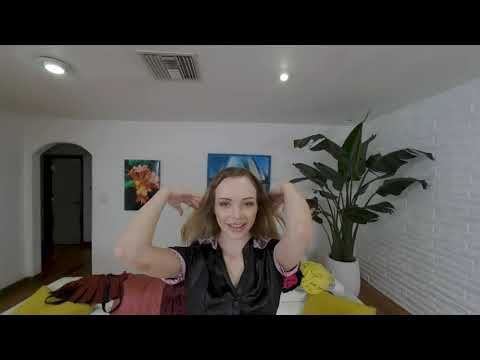A young woman, likely in her early to mid-twenties with light brown, thin hair, stands in a room with her arms bent at the elbows and hands near her head, as if caught mid-gesticulation or running her fingers through her hair. She is dressed in a black silk dress top that features pink chiffon ruffles at the edges of the short sleeves. The room has a mixed décor; directly behind her, the wall is regular white paint, while the right side features white brick. The background includes a doorway and a picture on the wall with pink and green floral elements, as well as another picture of a sailboat on an ocean. To the right, a large green plant in a white pot is visible, and the ceiling showcases two lights and a vent. Additional elements in the room include a yellow, pink, and maroon object, possibly on a table or the floor. Framing elements such as black rectangles are present at the top and bottom of the image, suggesting it might be a screenshot from a video, potentially for online content such as a YouTube tutorial.